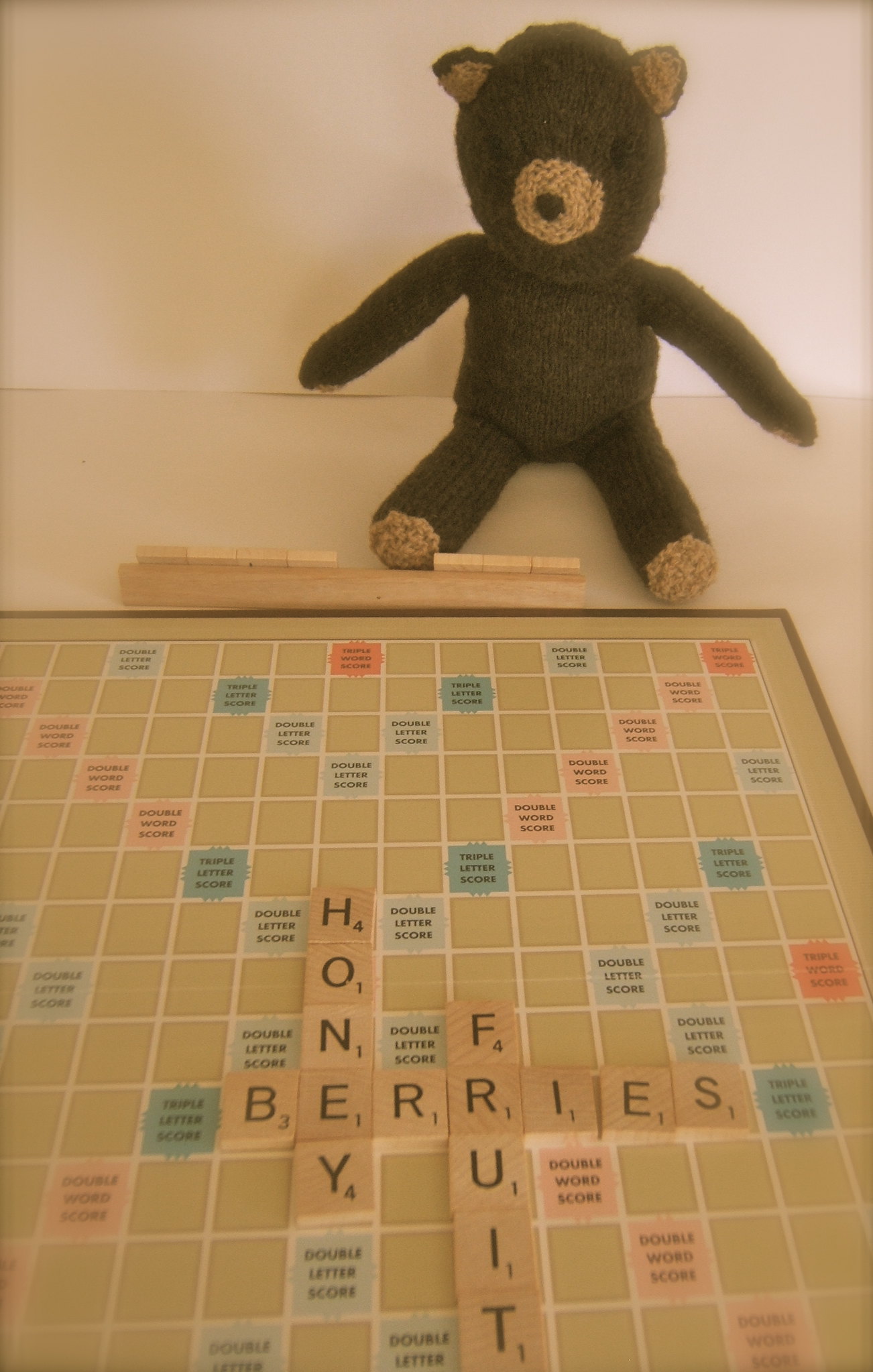This captivating photo showcases a whimsical Scrabble game setup in a pristine, white-walled, and white-floored room. The focal point is a vintage brown teddy bear, posed as if playing the game. In front of the bear, a wooden tile holder holds Scrabble tiles, arranged to mimic a typical player's strategic setup. The Scrabble board, a light brown base adorned with an array of colorfully shaded squares—ranging from light blue and dark blue to pink and orange—displays words like "honey," "berries," and "fruit." Detailed and humorous, this image uniquely combines a playful game scenario with the charm of a nostalgic toy companion.